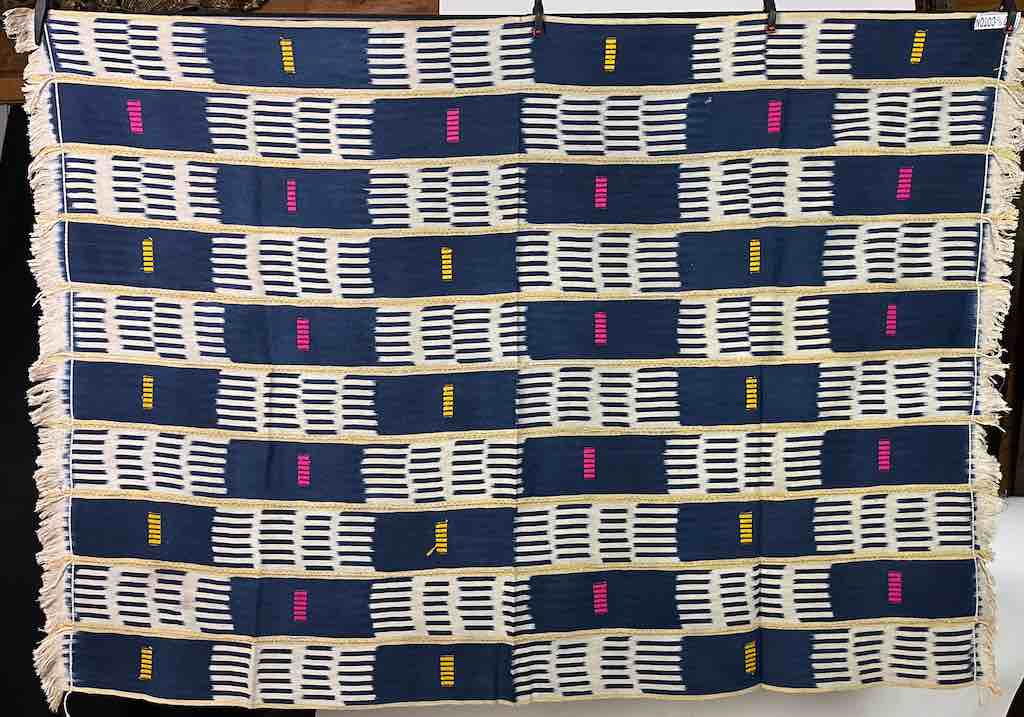The image features a patchwork-style quilt or blanket, displayed in a landscape orientation with a thin border running along the edge. The quilt is adorned with off-white tassels on both the left and right sides. It is held up by four slightly rusty metal clips at the top, which are unevenly spaced.

The patchwork design consists of ten rows and six columns of rectangular patches, creating a checkerboard pattern. The white rectangles are decorated with navy blue lines that form a partial plaid design, while the navy blue rectangles feature alternating center lines in yellow and pink. This alternating color pattern is consistent both horizontally and vertically throughout the quilt, with rows of navy blue rectangles containing yellow lines in the first, third, fifth, seventh, and ninth rows, and pink lines in the second, fourth, sixth, eighth, and tenth rows.

In the top right corner of the quilt, there is a small, sewn-on white label with blue text that is too small to read. The overall effect of the design is a striking and intricate plaid-like pattern, interspersed with colorful accents.